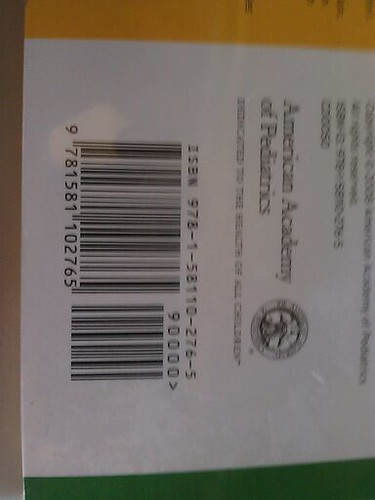This image appears to have been taken sideways, requiring rotation to discern its proper landscape orientation. It depicts the back cover of a book, identified by its visible barcode and ISBN. The ISBN provided is 978-1-58110-276-5, identical to the barcode number displayed. A smaller adjacent barcode bears the number 90000 (9-0-0-0-0) with a caret symbol above the ISBN. Positioned to the right in the sideways image, there is a partially legible text that reads "American Academy of Pediatrics." However, further details beneath this text are blurred and unreadable. Above "American Academy of Pediatrics," additional words are visible but indistinct.